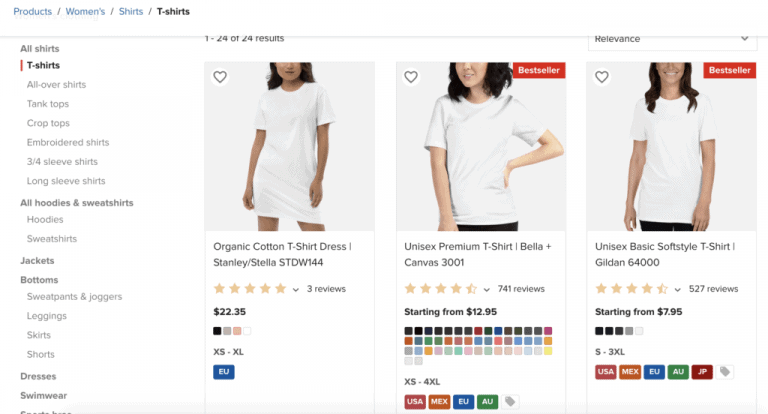This image depicts an e-commerce webpage showcasing a diverse array of clothing listings. The page is dedicated to women's apparel, featuring various categories such as t-shirts, all over shirts, tank tops, crop tops, embroidered shirts, full sleeve shirts, long sleeve shirts, hoodies, sweatshirts, and jackets. Additionally, there are options for bottoms including sweatpants, joggers, shorts, skirts, dresses, and swimwear. Highlighted on the page are three specific listings: an organic cotton t-shirt dress priced at $2.35, a unisex premium t-shirt (Bella + Canvas 3001) starting at $12.95, and a unisex basic soft style t-shirt available for $7.95. Each product appears with a detailed description and corresponding price, aimed at providing the customer with a variety of purchasing options.